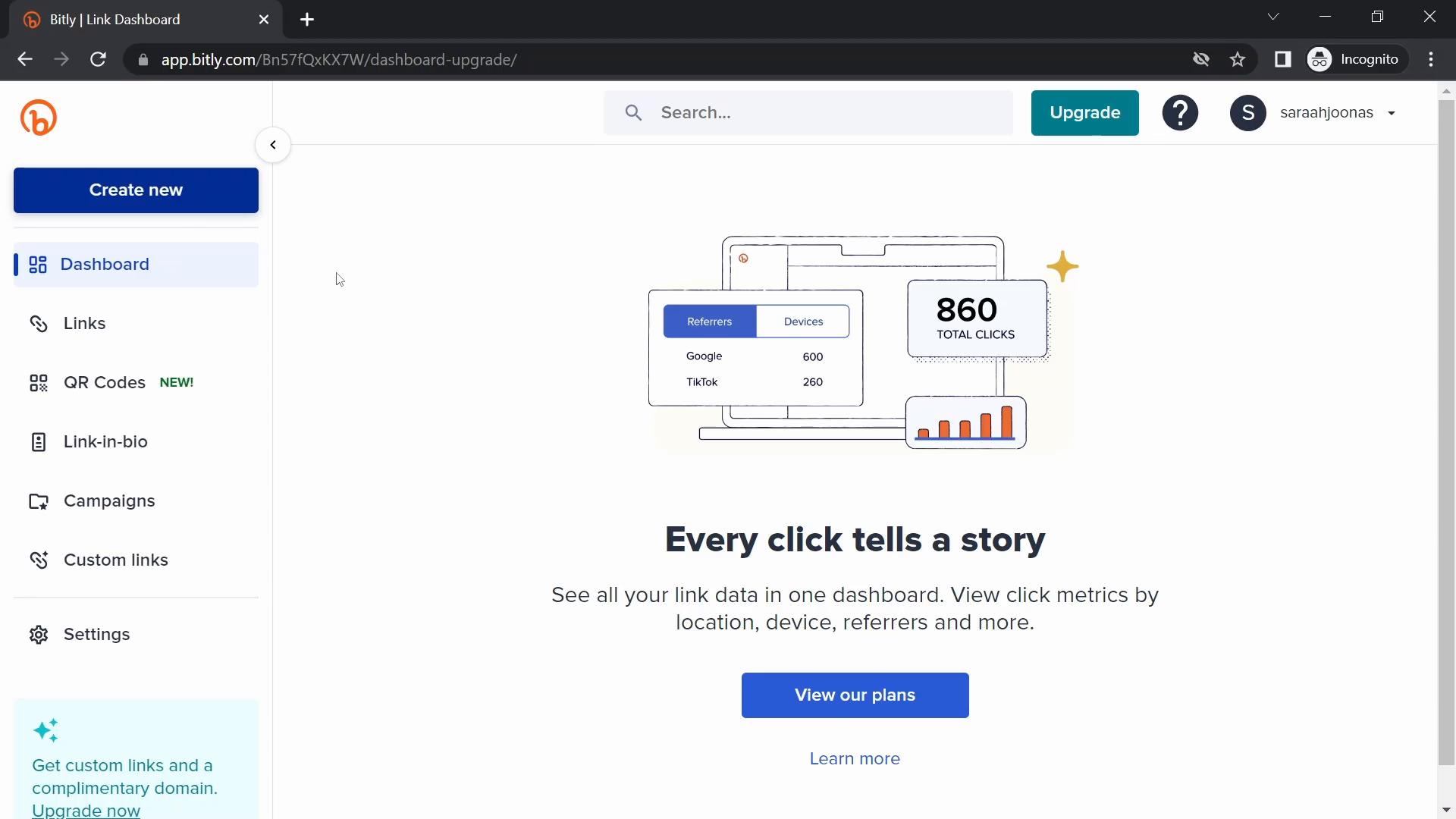The displayed webpage is the Bitly Link Dashboard, accessible via the URL "app.bitly.com/BN57FQXKX7W/dashboard-upgrades," which is shown in a black address bar with white text on a web browser. This browser has only one tab open.

Upon the Bitly page interface, there are several sections labeled: "Create New," "Dashboard," "Links," "QR Codes," "Link in Bio," "Campaigns," and "Custom Links." The Dashboard section is currently highlighted. The primary content displays an illustration of an open laptop with headings "Referrers" and "Devices." 

In the "Referrers" section, which is colored blue, the source data indicates "Google: 600" and "TikTok: 260," summing up to "Total Clicks: 860." Adjacent is the "Devices" section, presented in white.

A tagline below reads, "Every click tells a story. See all your link data in one dashboard," followed by a detailed description: "View clicks, metrics by location, device, references, and more." Finally, there are options for users to "View our plans" or "Learn more."